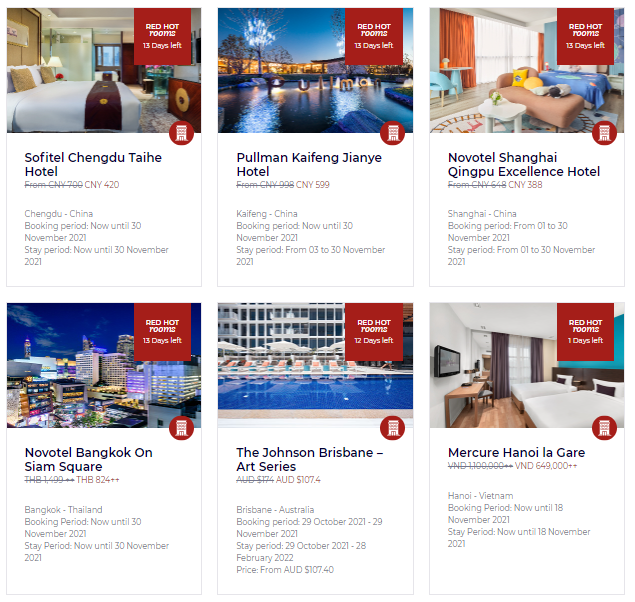### Detailed Descriptive Caption:

This screenshot appears to be from a travel or booking website showcasing various hotel deals under the promotional banner "Red Hot Rooms." The page lists details for several hotels, including their booking and stay periods, prices, and images of the hotel amenities and rooms.

1. **Sofitel Chengdu TAIHE Hotel**
   - **Price**: CNY 420
   - **Location**: Chengdu, China
   - **Booking Period**: Now until 30 November 2021
   - **Stay Period**: Now until 30 November 2021
   - **Image Description**: The image at the top features a luxurious hotel room with a large bed in the center, adorned with a white comforter. The photograph is overlaid with a text square that reads, "Red Hot Rooms 13 days left."

2. **Pullman Kaifeng Jianye Hotel**
   - **Price**: CNY 599
   - **Location**: Kaifeng, China
   - **Booking Period**: Now until 30 November 2021
   - **Stay Period**: 3 to 30 November 2021
   - **Image Description**: The next image shows a swimming pool illuminated at night, accompanied by the text, "Red Hot Rooms 13 days left."

3. **Novotel Shanghai Qingpu Excellence Hotel**
   - **Price**: CNY 388
   - **Location**: Shanghai, China
   - **Booking Period**: 01 to 30 November 2021
   - **Stay Period**: 01 to 30 November 2021
   - **Image Description**: This image showcases a brightly colored hotel room with the banner, "Red Hot Rooms 13 days left."

4. **Novotel Bangkok on Siam Square**
   - **Price**: THB 824
   - **Location**: Bangkok, Thailand
   - **Booking Period**: Now until 30 November 2021
   - **Stay Period**: Now until 30 November 2021
   - **Image Description**: Here, a stunning image of a cityscape at night is displayed with the caption, "Red Hot Rooms 13 days left."

5. **The Johnson Brisbane Art Series**
   - **Price**: AUD 107.40
   - **Location**: Brisbane, Australia
   - **Booking Period**: 29 October 2021 to 29 November 2021
   - **Stay Period**: 29 October 2021 through 28 February 2022
   - **Image Description**: This image shows a luxurious swimming pool with the label, "Red Hot Rooms 12 days left."

6. **Mercure Hanoi La Gare**
   - **Price**: VND 649,000
   - **Location**: Hanoi, Vietnam
   - **Booking Period**: Now until 18 November 2021
   - **Stay Period**: Now until 18 November 2021
   - **Image Description**: The final image features a hotel room with two large beds, labeled "Red Hot Rooms 1 day left."

Each hotel listing is accompanied by specific booking and stay periods, ensuring prospective travelers have all the necessary information to plan their trips.